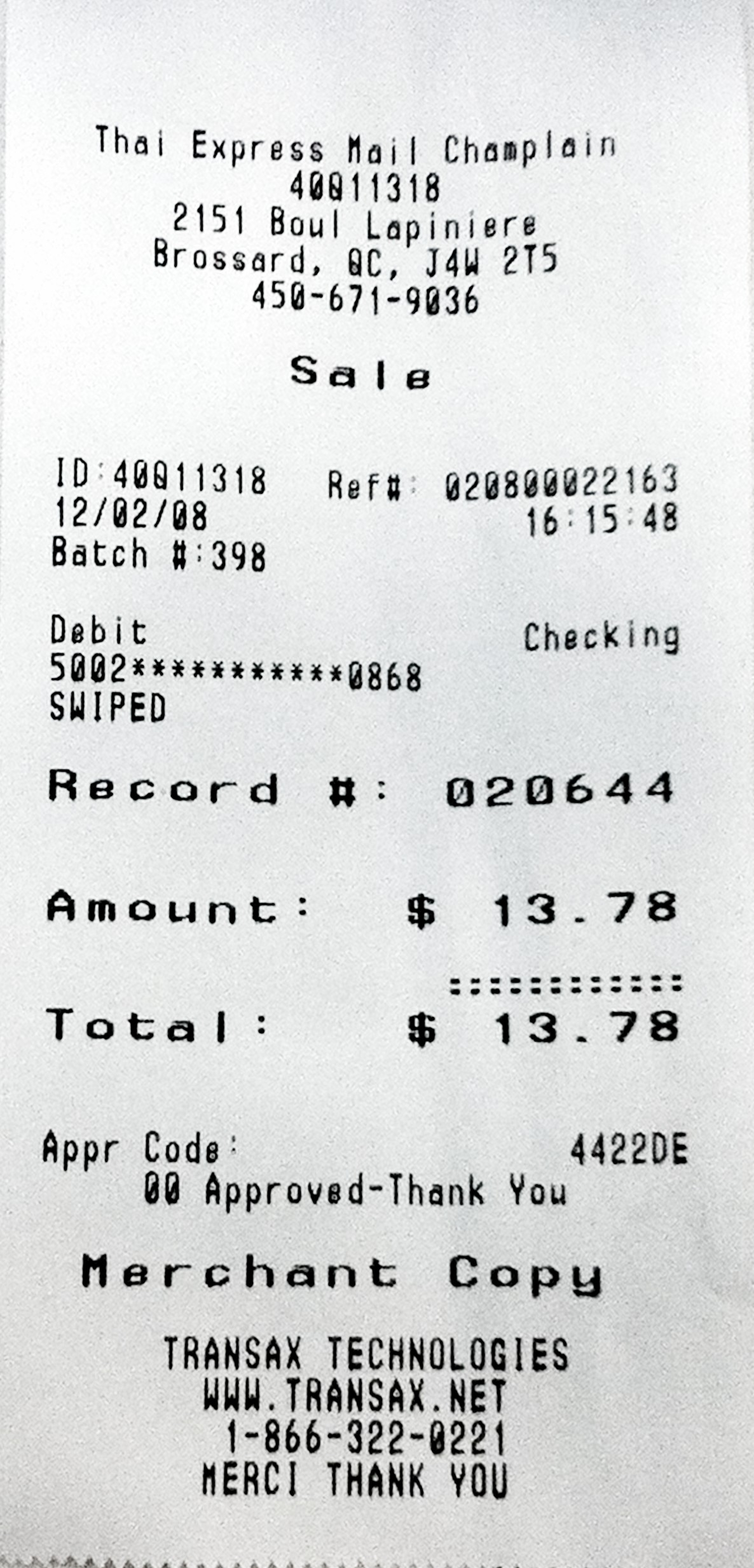The image depicts a standard-sized, horizontally-oriented white receipt featuring black print in various sizes. At the top, it reads "Thai Express Mail Champlain," followed by an identifier "400-113-18." Below this header is the address: "2151 Boulevard Lapinière, Brossard, QC J4W 2T5," and a contact phone number: "450-671-9036." The receipt notes the transaction category as "Sale" along with multiple identification numbers, including a record number "020644," an ID number, and a reference number. The transaction was processed on the date "12-208" at the time "16:15:48" and was paid using a debit checking card, specifically by swiping the card. The receipt displays part of the card number alongside another record number for the transaction. Both the amount and the total sum to $13.78 with no additional taxes applied. The approval code for the transaction is "4422DE," and it carries a note "Approved Thank You." At the bottom of the receipt, it indicates "Merchant Copy," the processing service "Transact Technologies," a website "www.transax.net," and a customer service phone number "1-866-322-0221." It ends with a bilingual "Merci / Thank You."